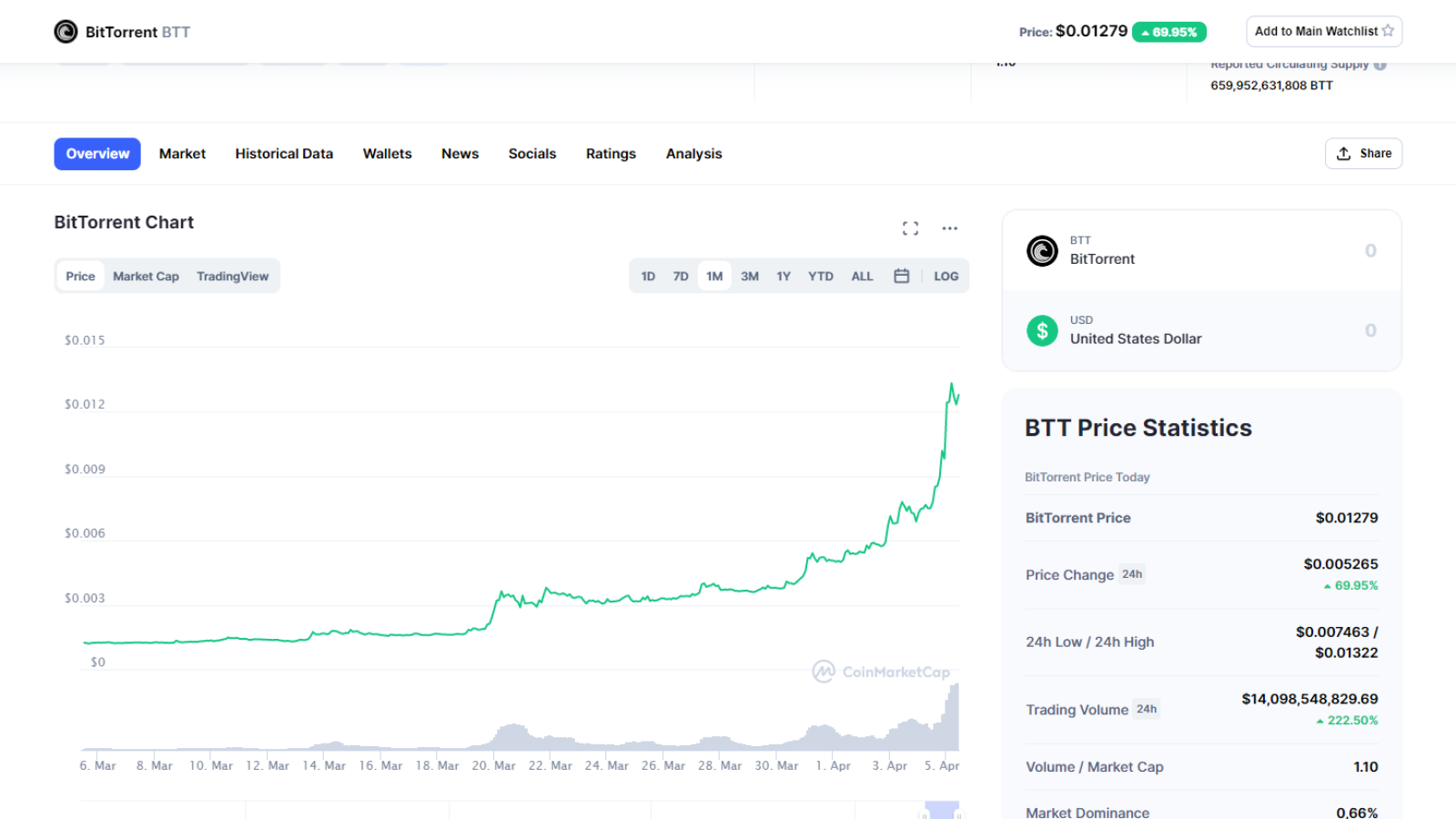**Detailed Description of the BitTorrent Price Screenshot:**

The image is a rectangular landscape screenshot from a laptop or desktop display. The background is predominantly white, and the interface shown belongs to BitTorrent, resembling a typical stock price chart.

**Header Section:**
- At the upper left corner, the BitTorrent logo is present, characterized by a black circle with shades of gray, and the word "BitTorrent" written in black font beside it. The logo is followed by "BTT" in gray, all capitalized.
- On the right side of the header, the word "Price:" is displayed, followed by the bolded price "$0.01279."
- Adjacent to the price, there's a teal green rectangular badge with rounded corners, featuring an upward arrow and the text "88.95%," though it is small and not easily legible.
- Next to this badge, another rectangular button with rounded corners and a white background outlined in gray contains the text "Add to Main Watch List" and an empty white star icon aligned on the right.

**Navigation Tabs:**
- Below the header, there are navigation tabs featuring options like "Overview," "Market," "Historical Data," "Wallet," "News," "Socials," "Ratings," and "Analysts," written in bold black font.
- The "Overview" tab is highlighted in white text against a medium blue background, signaling that it is currently selected.

**Chart Area:**
- Under the "Overview" tab, the title "BitTorrent Chart" is displayed.
- The main content of the image is the stock-like chart that occupies about 70% of the image's width.
- On the y-axis (left side), the price increments are marked in light gray starting from "$0.003" at the bottom and going up to "$0.015" in increments of $0.003, with an additional label for zero at the bottom, making a total of six price markers.
- The chart itself is represented by a friendly light green line. This line begins slightly above the $0 mark, indicating a starting price around $0.001, and remains relatively flat for roughly 40-50% of the chart's width before it begins an upward trajectory. The final 20% of the chart shows a notable spike, with the green line approaching the $0.015 mark in a jagged, non-smooth fashion.
- The x-axis at the chart's bottom lists dates, from "6 MAR" on the left to "5 APR" on the right, spaced approximately every two days.

**Sub-chart and Time Intervals:**
- Below the main chart, there's a smaller, darker gray chart that mirrors the larger one above, though its specific function isn’t clear.
- Above the green price change badge on the upper right of the chart, there are date headers for different time intervals: "1D," "7D," "1M," "3M," "1Y," "YTD," "All," and "Log." The "1M" (1 Month) option is highlighted.

**Statistics Panel:**
- The right panel, against a light gray background, provides several statistics under the heading "BTT Price Statistics."
- The first statistic lists "BitTorrent Price" with the same $0.01279 value.
- Subsequent rows include "Price Change" and other metrics, such as "Market Dominance," noted at "0.66%."

Overall, the image is densely packed with financial data and interactive elements, presenting a comprehensive view of BitTorrent’s price dynamics, similar to traditional stock market charts.